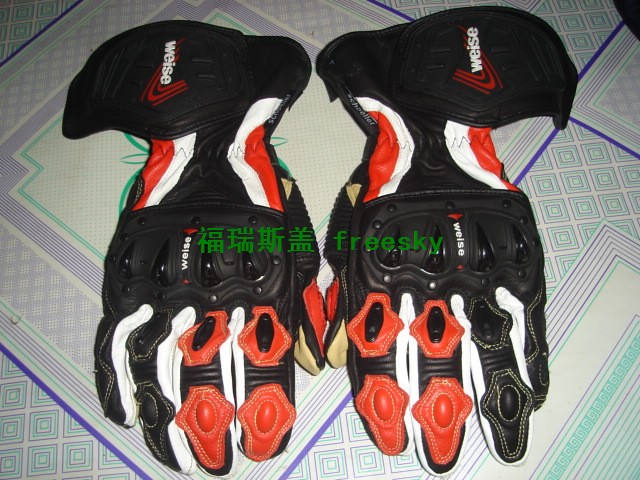This image depicts a pair of reinforced motorcycle gloves made by the brand Weisse (W-E-I-S-E). The gloves are primarily black with white and red accents. Notably, they feature stitched-on, red protective patches on the index and middle fingers, while the remaining fingers have black protective patches. These protective elements are arranged in two segments per finger: one near the bottom and another near the top. The knuckles are further protected by additional plastic coverings. The Weisse brand name is prominently displayed in white lettering across the knuckles and near the cuffs, along with green Asian script and the word 'Freesky' (F-R-E-E-S-K-Y) also in green.

The gloves are laid out side by side with the thumbs touching, fingers pointing downward, and wrists at the top of the image. They rest upon a colorful, patterned surface, which appears to be a quilt featuring a variety of colors including white, lavender, green, and light blue, with an intricate design that includes floral and diamond patterns.